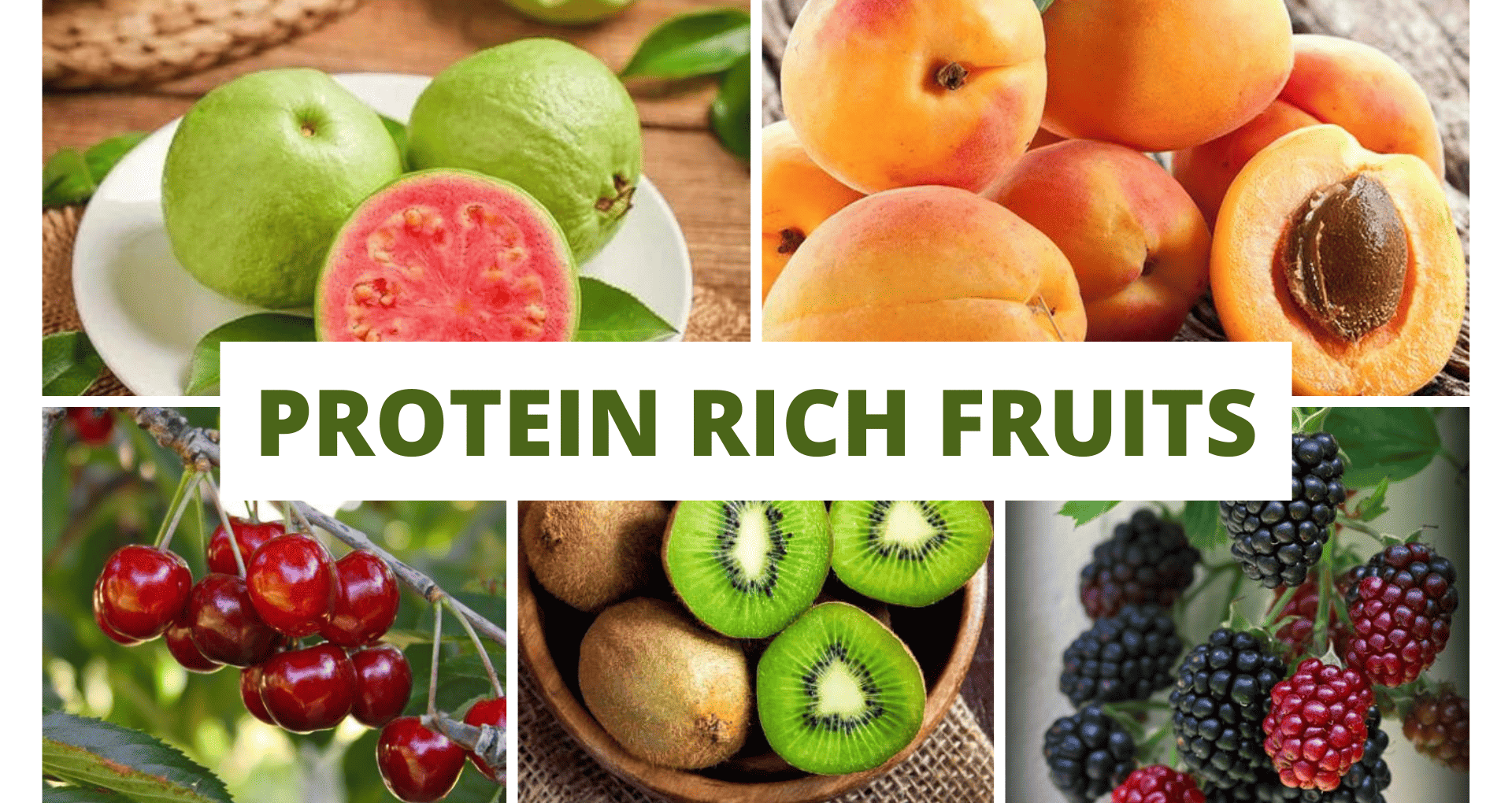The image is a meticulously arranged collage titled "Protein-Rich Fruits," suitable for a book cover or magazine feature. At the top left, there is a white plate with bright green guavas, one cut in half showcasing its pinkish-red interior, while green leaves adorn the plate. The top right displays a stack of apricots, including one cut open to reveal its orange flesh and seed. In the bottom left section, a cluster of black cherries rests on a brown stem. The bottom center features a bowl filled with brown, hairy kiwis, with three of them cut in half to expose their green insides, and lying on a brown cloth. Finally, the bottom right corner shows an array of black and red berries, including eleven blackberries and two reddish ones, some still attached to green stems. The overall presentation emphasizes the vibrant colors and varied textures of these protein-rich fruits, captioned with "Protein-Rich Fruits" in green text on a white bar at the center of the image.